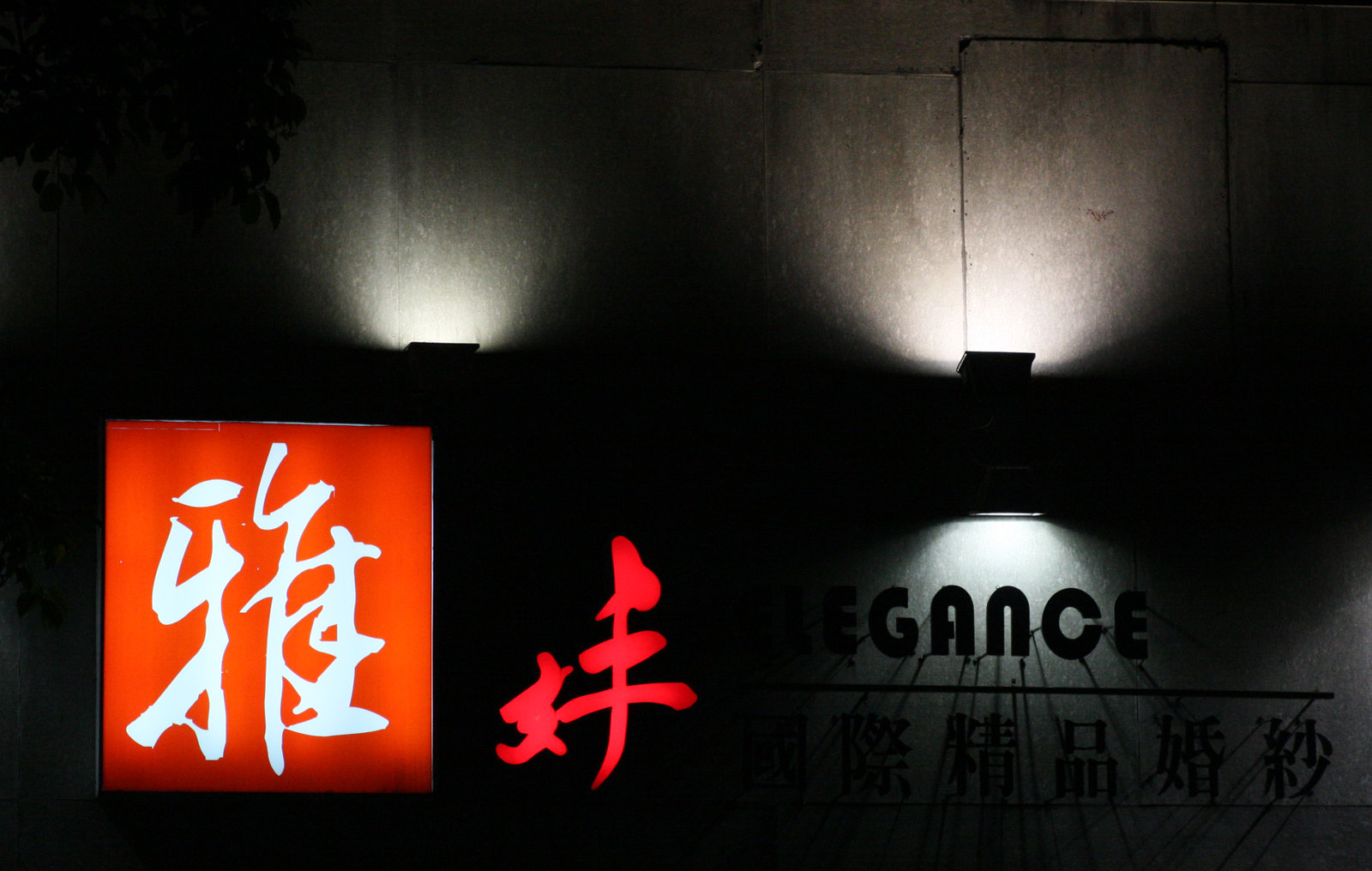This image is a dark, atmospheric nighttime photograph of a building's exterior wall, likely part of a business such as a club or restaurant. The structure appears to be made of heavy concrete or stone in large slabs. There are three floodlights creating a dramatic spotlight effect: two on the left and right sides shining upwards, and one centrally placed shining downwards, forming an inverted horseshoe shape of illumination. In the bottom left corner is a red illuminated box with a white Japanese character inside. Adjacent to this box, closer to the center, is another red Japanese character. To the right of these characters is a section illuminated by the downlight, where partially visible English letters can be seen, likely spelling 'ELEGANCE.' Beneath this word are additional black Japanese characters, faintly visible in the spotlight's shadow. The overall dark setting highlights the illuminated signage and characters, creating a vivid and mysterious ambiance.